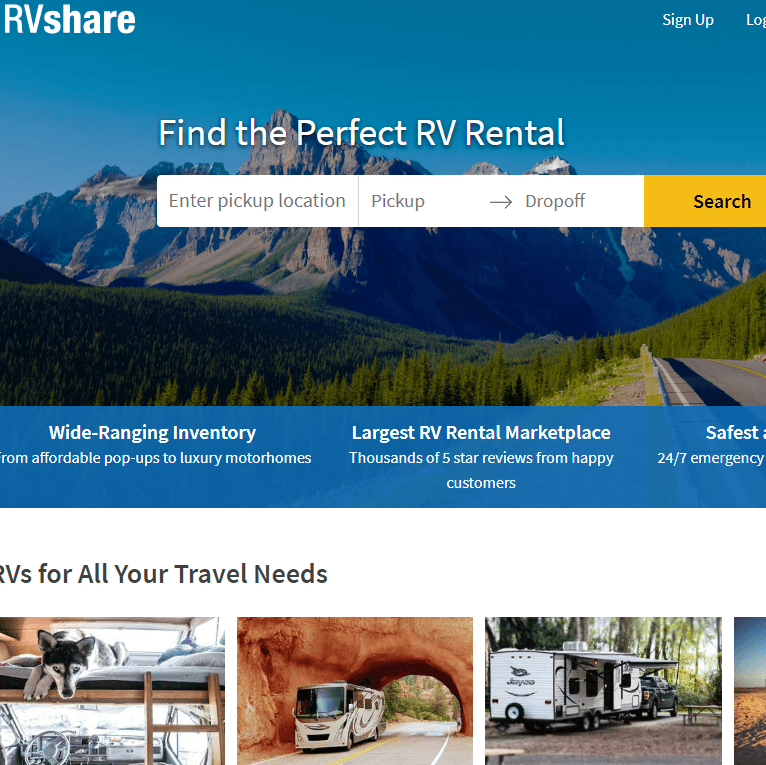The image features a promotional banner for RVshare, an RV rental marketplace. At the top, a large blue box prominently displays the RVshare logo in the upper-left corner. Adjacent to the logo, options for "Sign Up" and "Log In" are clearly visible. The central message reads, "Find the Perfect RV Rental," accompanied by fields to enter a pickup location, pickup and drop-off dates, and a search button.

The background scenery is breathtaking, showcasing beautiful mountains, lush green grass, vibrant trees, and a winding highway. Beneath the scenic view, another blue box highlights key features of RVshare: a wide-ranging inventory from affordable pop-ups to luxury motorhomes, the claim of being the largest RV rental marketplace, and assurance from thousands of five-star reviews by satisfied customers. It also emphasizes the safety aspect with 24/7 emergency support.

On a white backdrop, the phrase "RVs for All Your Travel Needs" stands out, providing additional context and reassurance. Adjacent to this text are three distinct images: the first depicts a cozy loft scene with a cute dog, the second shows a long RV resembling a bus navigating through a tunnel, and the third captures an RV set up at a serene camping spot.

This detailed and visually appealing banner effectively conveys the excitement and reliability of renting an RV through RVshare.